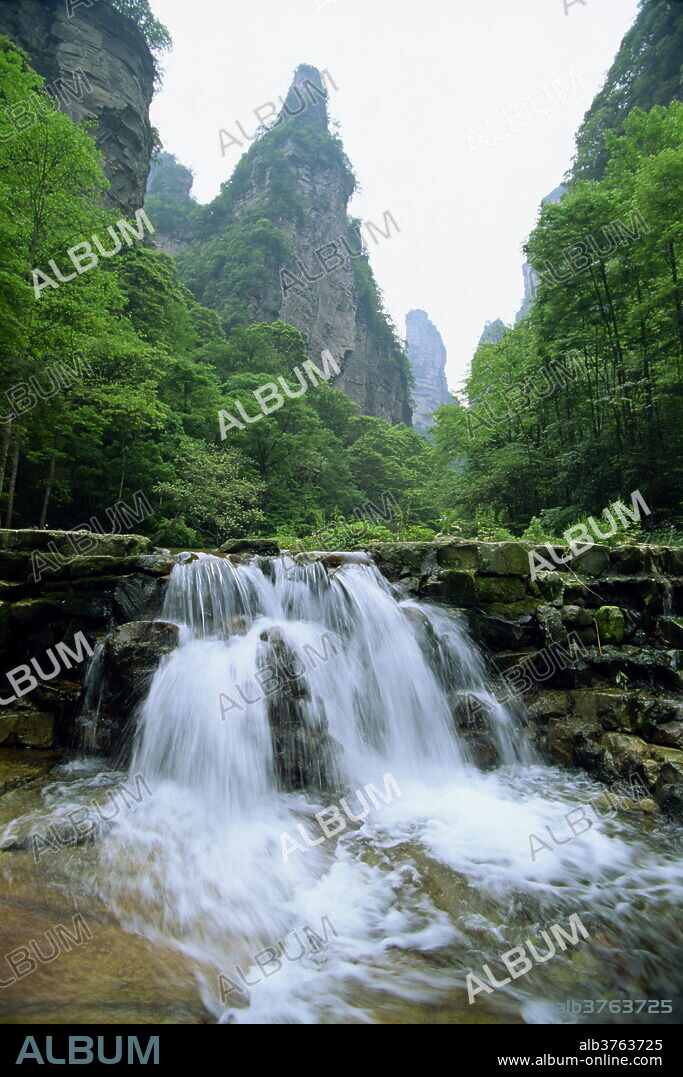This vertical rectangular image, possibly an album cover or advertisement for where to listen to an album, captures a serene outdoor scene centered around a small, flowing waterfall. The waterfall cascades down a moss-covered, stone wall of dark green rock into a shallow pool, rich with white, frothy water. Above the waterfall, the landscape extends into lush, verdant trees and tall rock structures partially obscured by vegetation, set against a bright, gray sky. The photo is marked with the word "album" in white and gray across the image, giving it a distinct, watermark-like appearance. At the bottom, a black band spans the width of the image with "album" written in gray letters on the left and, on the right, the text "ALB3763725" alongside the website "www.album-online.com," adding to the commercial and promotional feel of the image.